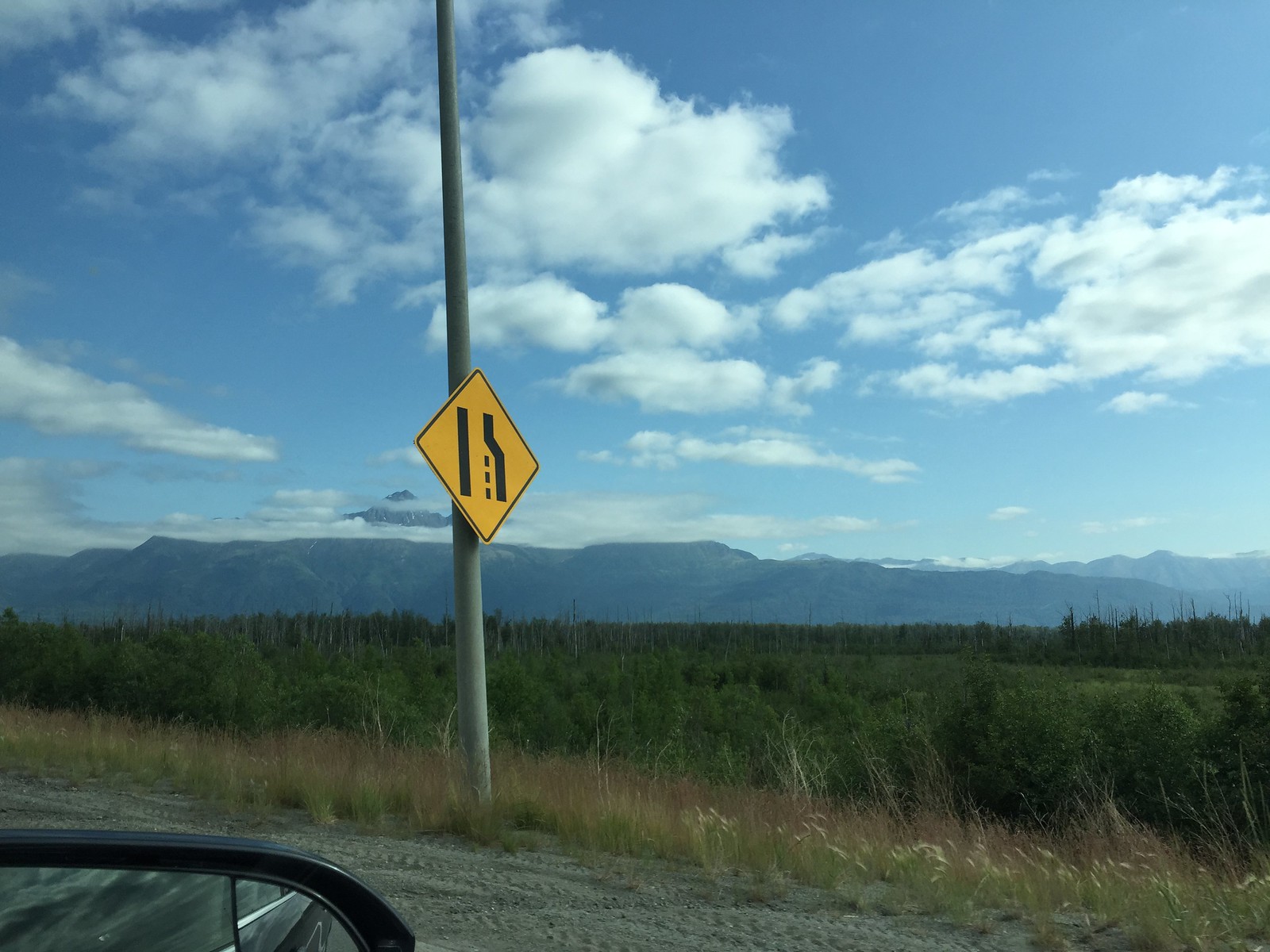A scenic view of a countryside dirt road is captured through the side mirror of a black car. The road's shoulder appears well-trodden with visible tire tracks. Dominating the foreground is a large, silvery pole with a diamond-shaped traffic sign indicating a solid line for straight travel and a dashed line suggesting a merging lane. Above, the sky is a vibrant blue filled with scattered clouds. The distant background boasts majestic mountains, while closer to the road, a sprawling green field dotted with evergreen trees is visible. Along the edge of the road, tall, dry grass interspersed with colorful wildflowers adds a rustic charm to the landscape.